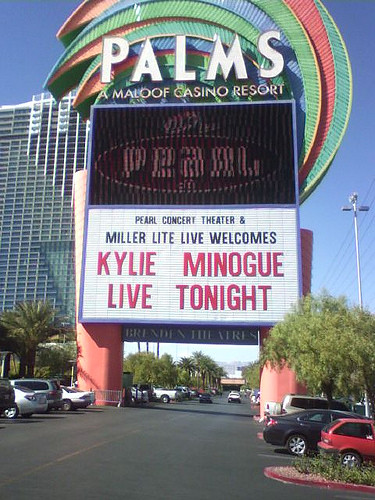This outdoor daytime photograph showcases the Palms, a Maloof Casino Resort, with a vivid, multi-colored sign featuring green, red, and yellow curved shapes resembling a palm. At the top of the sign, "Palms" is prominently displayed, indicating the resort name. Below that, an electronic screen reads "Pearl," and further down, a marquee in red lettering announces, "Pearl Concert Theater and Miller Lite welcomes Kylie Minogue, live tonight." The setting includes a gray asphalt parking lot beneath the sign, filled with various cars, including a red one, a black one, and a few white ones. To the left of the sign stands the casino's towering multi-story building, which appears to be at least 15 stories high. A light tower is seen to the right of the sign, all set against a backdrop of a clear, blue sky.